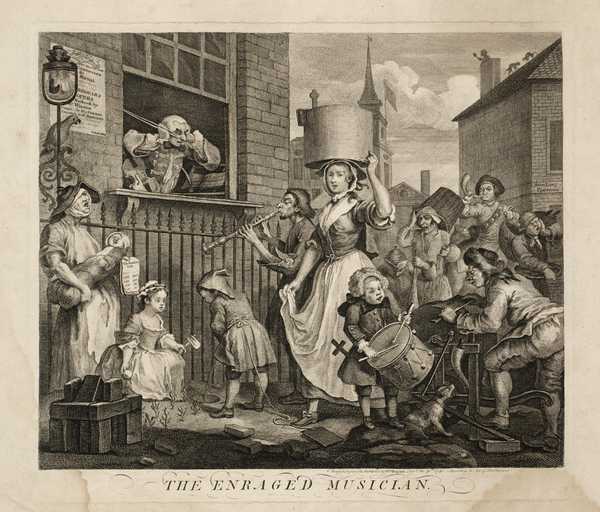The image is a detailed vintage cartoon drawing that appears to be set in a bygone era, characterized by its black and white illustration on creamy colored paper. The drawing, titled "THE ENRAGED MUSICIAN" as written in capital letters and italics within a beige colored frame, displays a bustling street scene with a variety of characters. 

In the center, a prominently featured woman in a dress and apron is lifting a large pot or barrel over her head. Beside her, a young boy equipped with a drum and possibly a cross or sword at his side, plays the drums, with a dog at his feet. The scene is lively with numerous individuals of different ages and genders engrossed in various activities. 

The background includes a man blowing a horn, another man playing the flute, and several other people with musical instruments like trumpets and barrel drums. To the left, a brick building stands with an open window, from which a man in an old-fashioned wig and fancy coat is visible, squeezing his hands against his ears in apparent distress due to the cacophony below.

An older woman is depicted holding a crying baby under a street lamp, further adding to the scene's vibrancy and chaos. This dynamic street scene captures the essence of a lively, yet disorderly musical ensemble moving across the image from right to left, encapsulating the title’s sentiment.